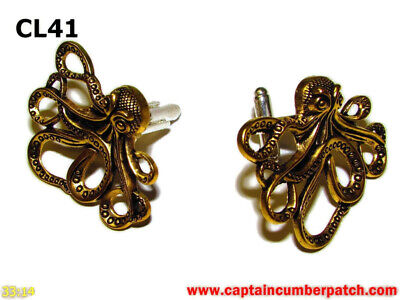This is a detailed, close-up, color photograph of a pair of intricate brass or gold earrings, possibly octopus-themed doorknobs, oriented in landscape. The background is a clean, unbroken white surface, which highlights the craftsmanship of the earrings. Each octopus features a rounded head with two prominent eyes and numerous intricately curled tentacles wrapping in various directions, exemplifying a high level of detail and design, possibly wire or filigree work. They are lying side by side, with the left one slightly angled to the left and the right one facing to the right. Behind each earring, partially visible, is a small cylindrical post designed for attachment. In the upper left corner of the image, the text "CL41" appears in black. Below the left earring, there's the number "33 By 1 4" in yellow, although it's partially indistinct. In the lower right corner, the red text reads "www.captaincumberpatch.com," suggesting that this image serves as an advertisement for these highly ornamental items. The photograph employs a realism style common in product photography.